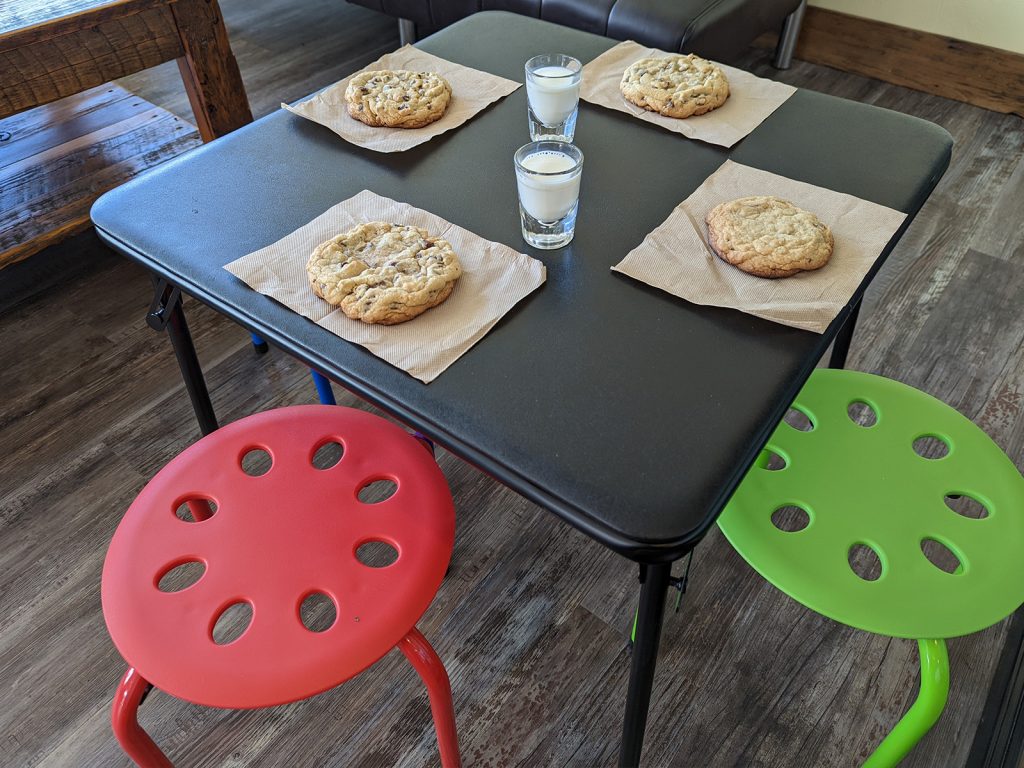The image depicts a small, black, square folding table set up indoors, positioned with a corner facing the viewer. The table is surrounded by three stools: a red stool on the left, a green stool on the right, and the partially visible legs of a blue stool in the background. The table features four brown paper napkins placed at each side, each bearing a large, homemade-looking chocolate chip cookie that almost matches the height of the napkin. Centrally positioned on the table are two glasses of milk, arranged diagonally to align with the table's orientation. The setting is within a room with wooden paneling on the floor, and there’s a suggestion of a leather couch and possibly a coffee table in the background, adding to the cozy, living room ambiance.